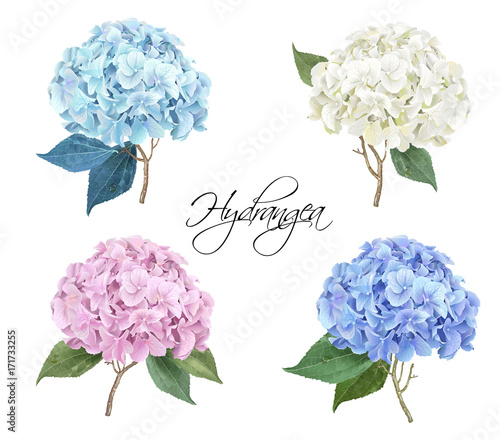This Adobe stock image features a beautifully arranged quadrants layout, each showcasing a distinct hydrangea bloom on a plain white background. The hydrangeas are of similar size, each occupying its own quadrant. In the upper left, a sky-blue hydrangea displays aqua marine blue leaves. The upper right corner features an off-white hydrangea, accompanied by green leaves. The lower left quadrant presents a medium pink hydrangea with three green leaves, while in the lower right, a purpley blue hydrangea is adorned with green leaves. Each hydrangea emerges from a brown stem. "Hydrangea" is elegantly written in cursive handwriting in black at the center of the image, and the image is marked by a watermark that reads "Adobe stock.” Additionally, a vertical label in the bottom left corner says "Adobe stock" followed by a 10-digit number, also in black writing.